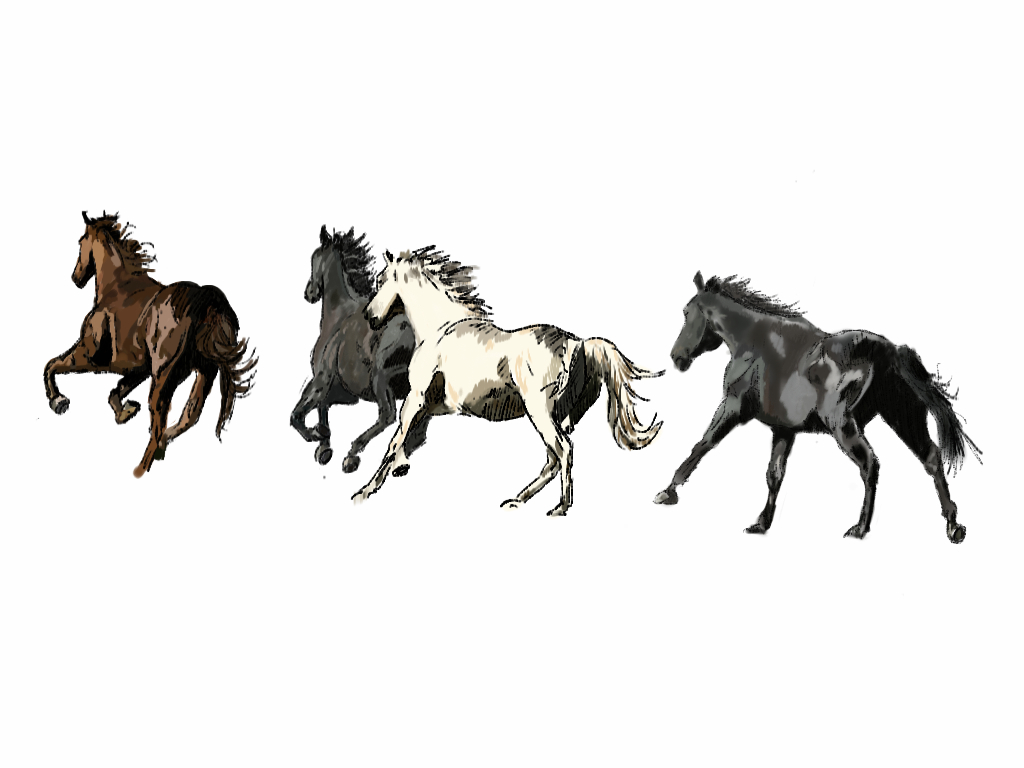This detailed colored sketch, created with ink outlines and art markers on white paper, depicts four horses galloping energetically from the bottom right to the top left corner of the image. The horses are in motion, their manes and tails flowing behind them as they run. Leading the group is a brown horse, followed by a white horse and two black horses. The white horse is positioned slightly ahead of the first black horse, creating a dynamic perspective. The last black horse appears to be just lifting its legs, preparing to fully join the others in their spirited run. The horses are outlined with precise detail, particularly noticeable in the white horse, and there is no background to the image, emphasizing the vibrant action of the galloping horses against the stark white backdrop.